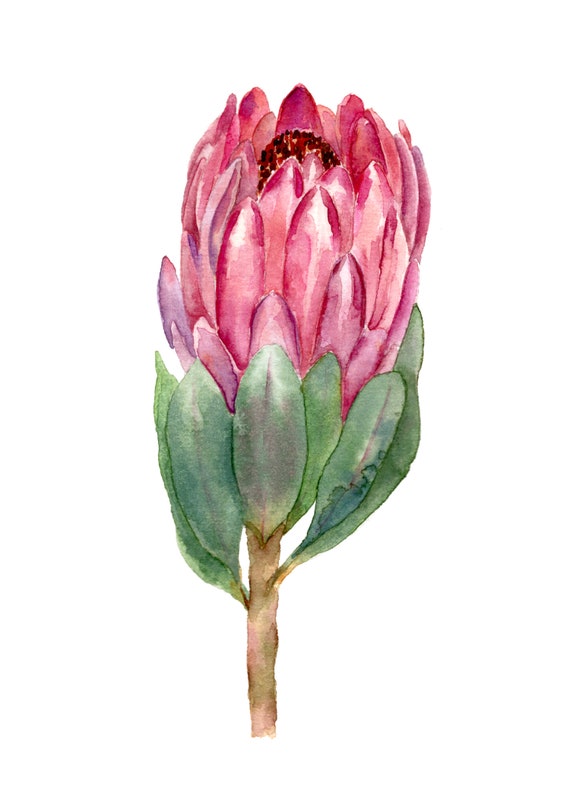This watercolor painting depicts a close-up of a beautiful flower that is not yet fully bloomed, appearing as if it’s closed in for the night. The flower, which resembles a mum, features an array of vibrant colors: the petals are a blend of dark pink, wine, and purple hues with white highlights, while a dark red and spotty pod, possibly consisting of stamens tipped with a brownish-orange color, peeks from the center. The focal point of the artwork is the flower’s bloom, which is complemented by oval-shaped green or green-gray leaves that fold upright, cradling the blossom. A brown stem supports the flower, which is positioned centrally and tilts slightly to the right. The painting is set against a stark white, transparent background without any text, signature, or additional borders, emphasizing the delicate and intricate details of the bloom and its surrounding leaves.